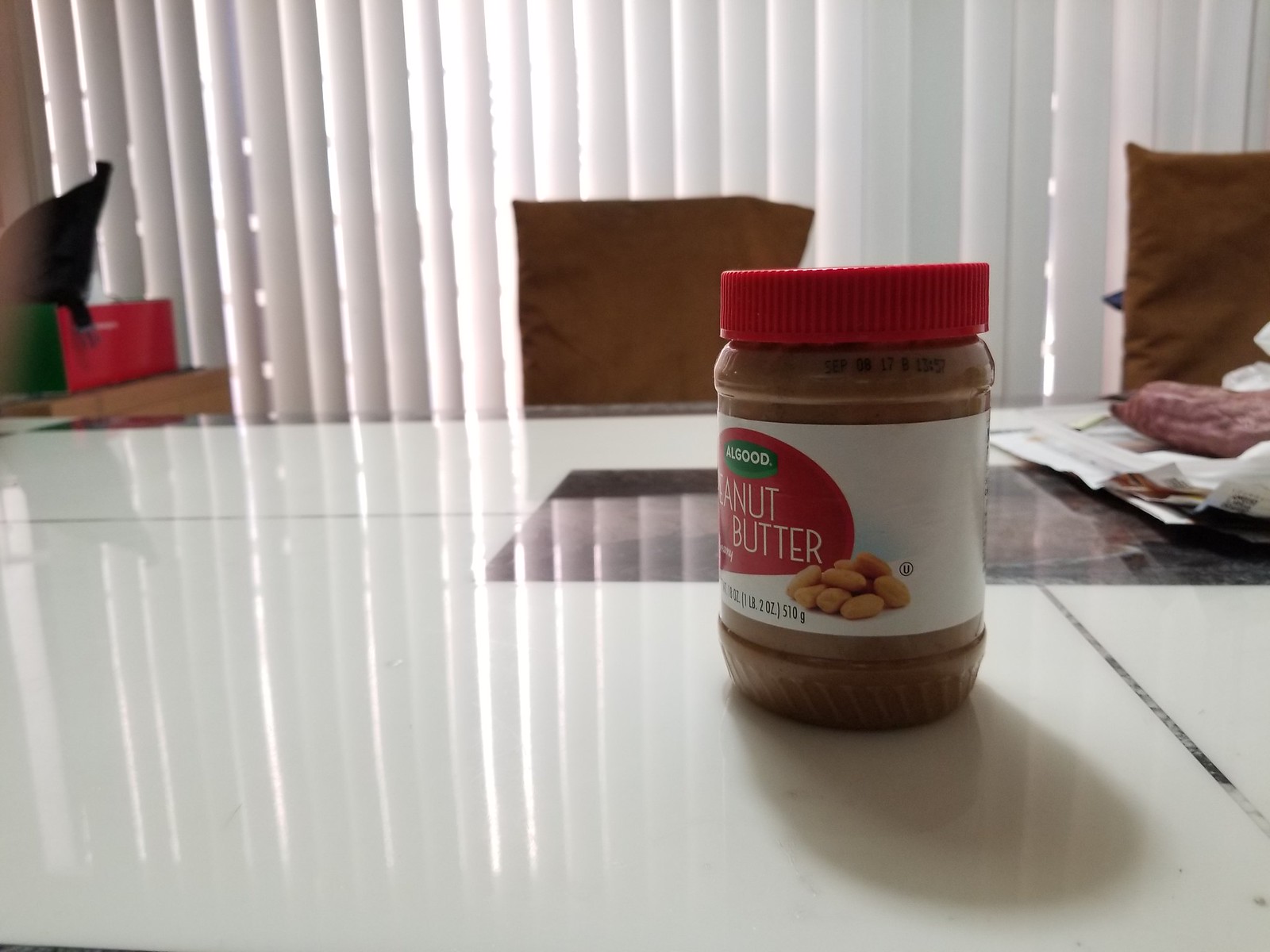The photograph captures a glossy white, glass-topped dining table with a prominently placed jar of peanut butter in the foreground. The jar, made of transparent plastic, is full and sealed with a red, ribbed screw lid. The label, which wraps horizontally around the jar, features a green geometric shape with white text indicating the brand "All Good." Another visible detail on the label includes the words "butter" with "peanut" partially obscured as it wraps around the side, and a small graphic of a pile of peanuts at the bottom right. A faint, black date and time stamp is visible around the neck of the jar, though it's too blurred to read clearly.

The background reveals two high-back dining chairs with medium-brown fabric coverings. Between the chairs, vertical window blinds let streaks of sunlight filter through, casting reflected light onto the glossy table surface. There also appears to be a burgundy inset square in the center of the table, adding distinct contrast to the white glass top. In the back left corner of the image, a red and green box is visible, perched on a wooden ledge, suggesting a hint of lived-in warmth amidst the otherwise clean and orderly setting.